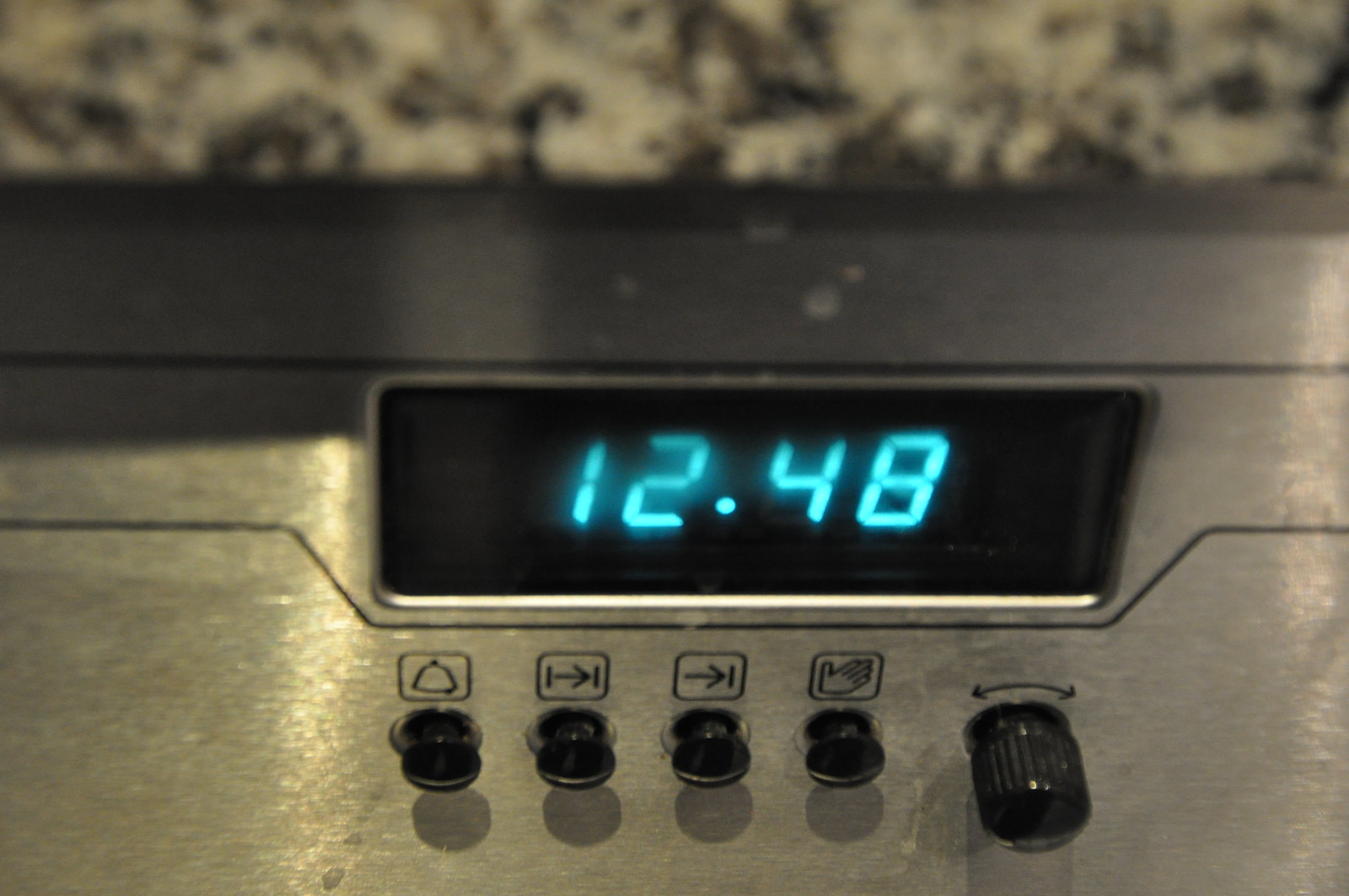Detailed Caption: 

This image showcases a digital clock mounted above a vent, possibly serving as a part of a larger control panel. The clock displays the time "12:48" with a single dot separating the hours and minutes. The entire setup is encased in a slightly tarnished silver surface, which exhibits some noticeable spots and smudges, adding a used, industrial feel to the scene. The image quality is a bit blurred, obscuring finer details.

Beneath the digital display, there is a large, circular knob prominently featuring left and right arrow indicators, suggesting it can be turned to adjust settings. Accompanying this primary knob is an array of several other controls:

1. A dial with traditional clock hands, accompanied by a knob for manual adjustment.
2. A control that moves to the right and is marked by a single vertical line positioned before the arrow.
3. Another control moving rightward, flanked by vertical lines on both the left and right, with the arrow situated between them.
4. Additionally, a control marked by a bell symbol, likely indicating an alarm or alert function, also featuring a mechanism for adjustment, either via twisting or pulling.

Each of these controls is equipped with knobs, contributing to the intricate and purposeful design of this multi-functional timekeeping and control device.